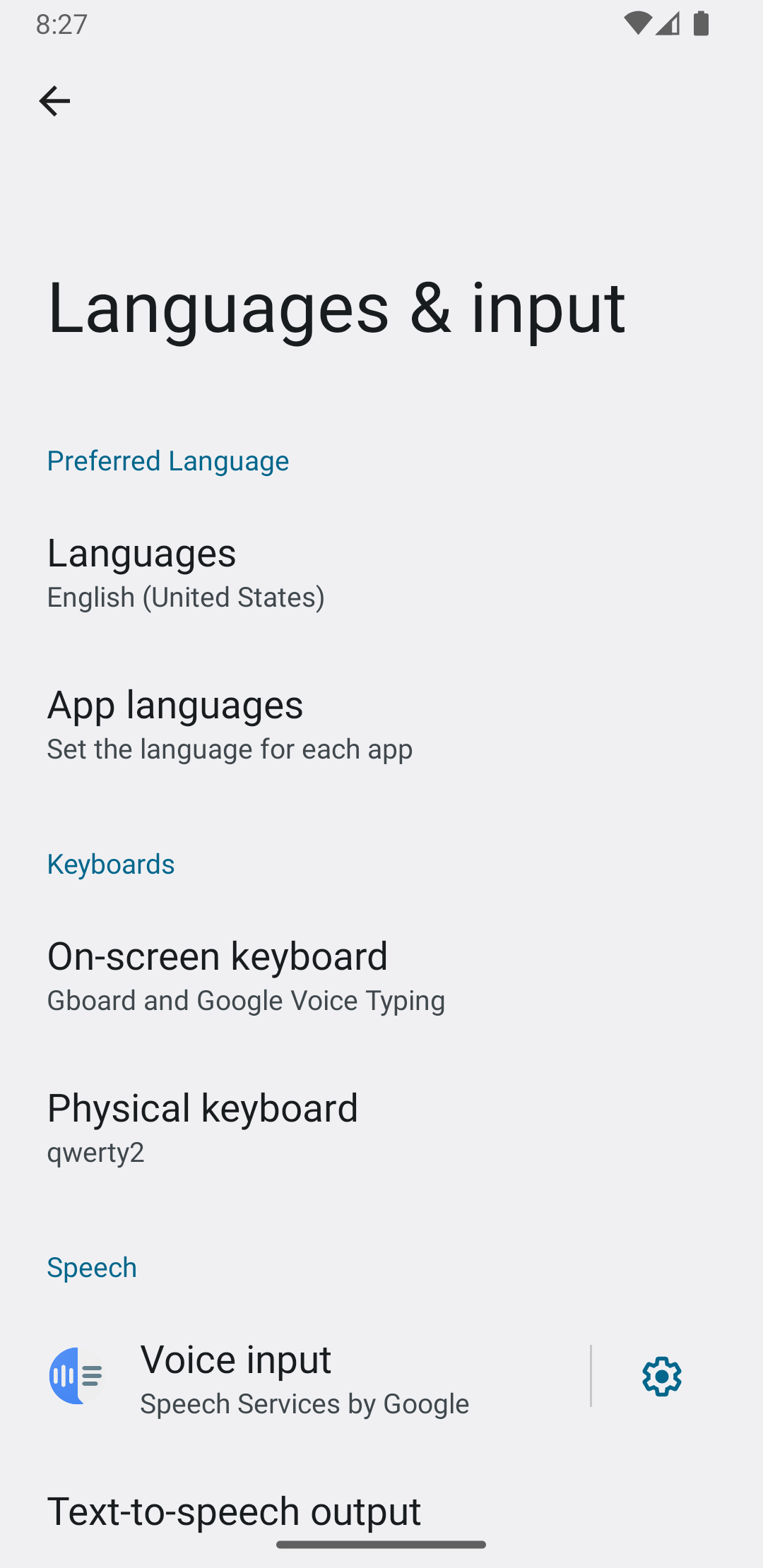This screenshot displays a smartphone screen captured at 8:27 p.m., showcasing a full battery and strong signal strength. The image presents the "Languages & input" settings menu against a light gray background. 

At the top, the title "Preferred language" is highlighted in blue. Below this, the "Languages" section reveals "English (United States)" as the selected language. 

Following this is the "App languages" section with a note indicating it allows users to set languages for individual apps.

Next, the "Keyboards" section is divided into two parts:
1. "On-screen keyboard" which includes options like "Gboard" and "Google voice typing".
2. "Physical keyboard" labeled as "QWERTY 2".

Further down, the "Voice input" option is managed by "Speech services by Google" with a teal settings icon adjacent to it. The final section is "Text-to-speech output," separated by a black line at the bottom of the screen.